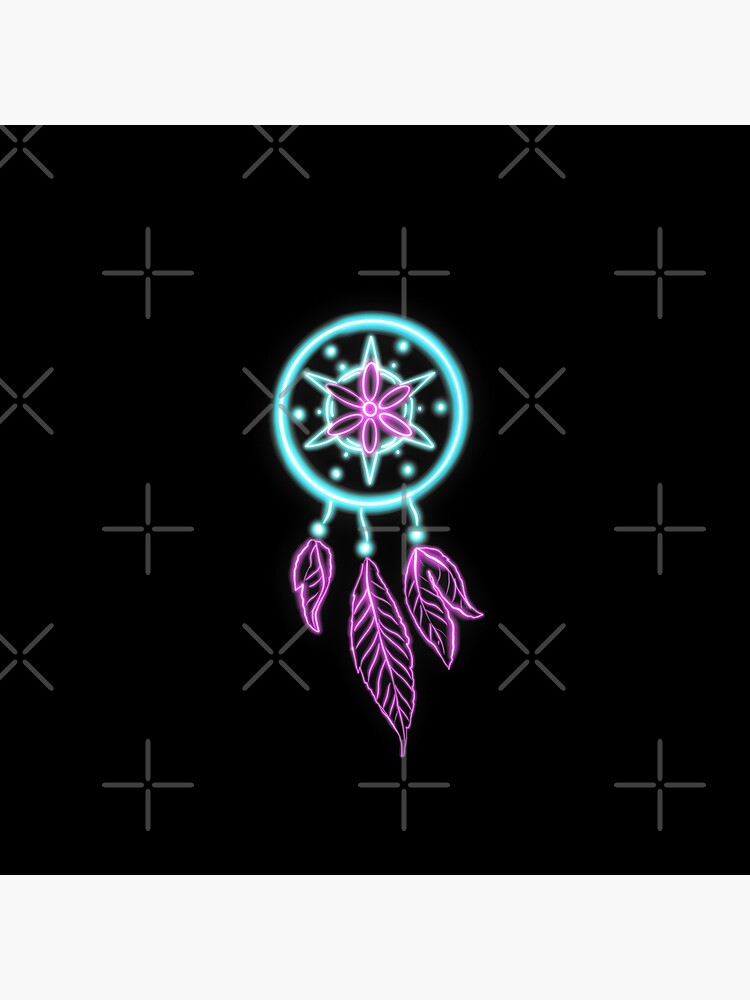The image appears to be a computer-generated or animated drawing with a completely black background. In the background, there's a detailed pattern of light gray X's and crosses, organized in alternating lines — three X's followed by three crosses, repeated multiple times for a structured look. The centerpiece of the composition is a vibrant neon dreamcatcher. The outer circle of the dreamcatcher is a bold teal, and it contains intricate details like a six-pointed star and small dots. Surrounding the interior star is a light purple hue. Hanging from the bottom of the dreamcatcher circle are multiple decorative elements: three short strings adorned with beads, and beneath them, three feathers that are a striking neon purple. The entire scene combines traditional dreamcatcher elements with a modern neon aesthetic.